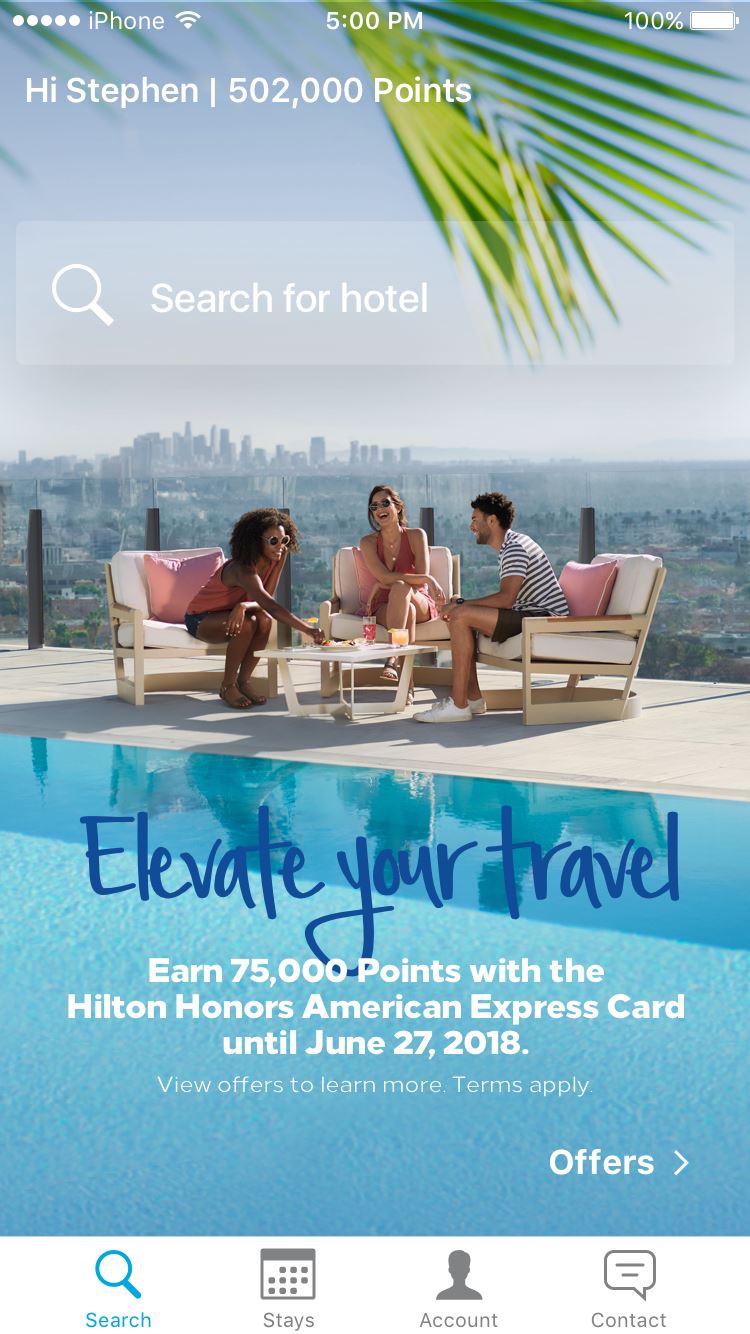In the top left corner of the image, there are five circles next to an icon that appears to resemble the letter "I," followed by the capital letter "P." All the Wi-Fi signal indicators are white. In the center of the top, the time is displayed as "5:00 PM." On the right side, "100%" is displayed, likely indicating full battery charge. 

Below this, in white text, it reads "Hi Steven" with a vertical line descending from it. The text then continues with "502,000 points," also in white, followed by a capital "P." There is a transparent rectangle featuring a white magnifying glass icon and the word "Search" with a capital "S," followed by "for hotel."

At the bottom of the image, in blue text, it says "Elevate your travel." Below this, in white text, it reads "Earn 75,000 points with a Hilton Honors American Express card until June 28th, 2008, learn more terms apply." Additionally, on the right side, there is an indicator for "offers" with an arrow point next to it.

Underneath this section, there is a blue magnifying glass icon adjacent to the word "search" written in blue. The phrase "stays in contact" is mentioned as well.

The background picture shows three people sitting on beige-colored chairs with pink pillows, gathered around a white table with drinks and some plates of food, positioned next to a pool.